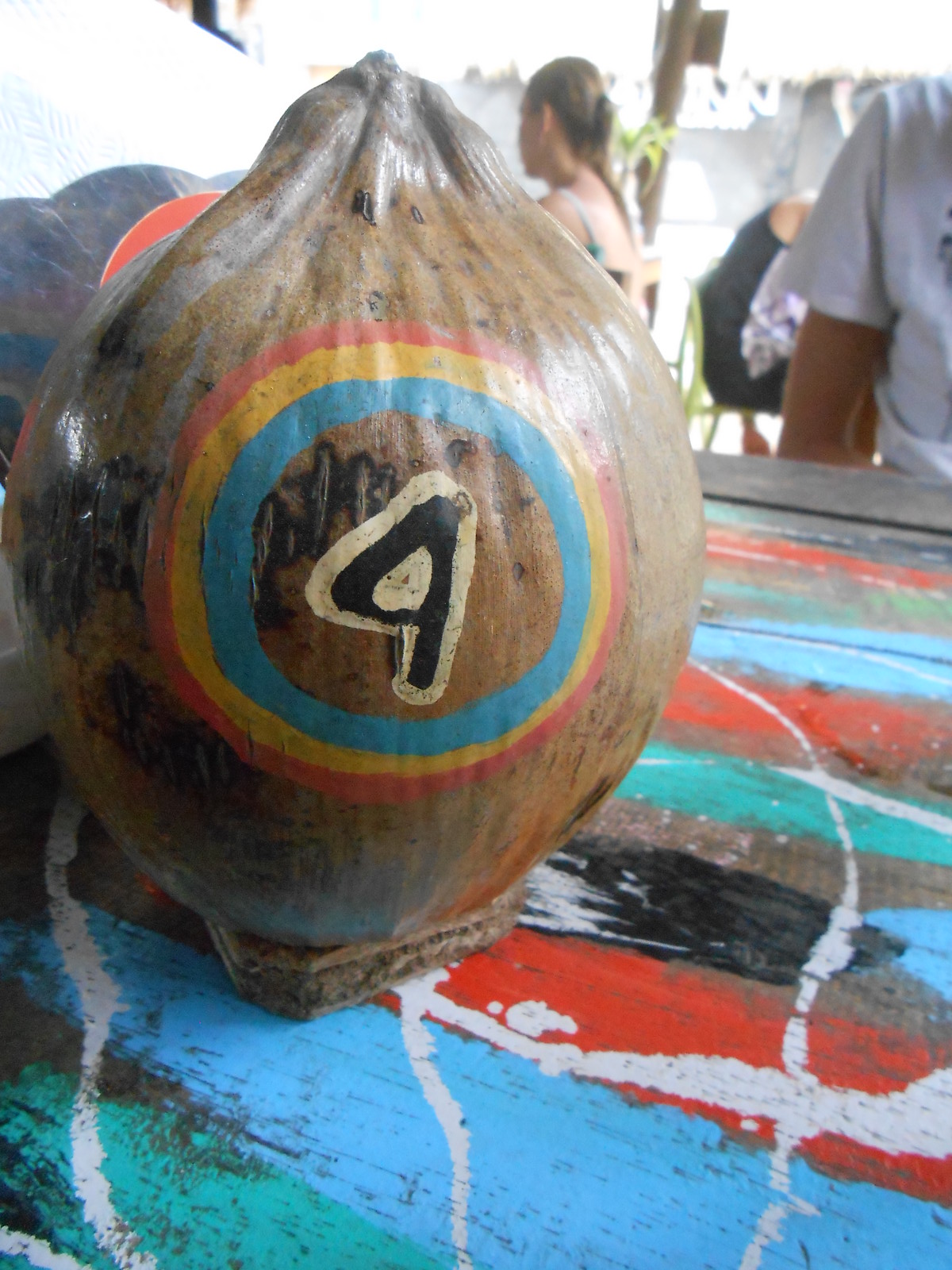In this detailed photograph, the focus is on a close-up of a large, round brown object that strongly resembles a coconut but could potentially be a carved wooden item. The object's surface, hard and shiny, features a distinctive painted design in the center: a blue circle encircled by a yellow ring, followed by a red ring. At the center of these concentric circles, the number four is prominently painted in black, outlined with white. This striking object is placed on a vividly colorful table, painted in stripes of teal, blue, red, black, and white. In the background, there is the partial view of a person in a short-sleeved white shirt, suggesting the scene might be set in an outdoor or café-like environment. Also visible is a woman with light brown hair tied into a ponytail, seated at another table, adding to the lively ambiance of the setting.